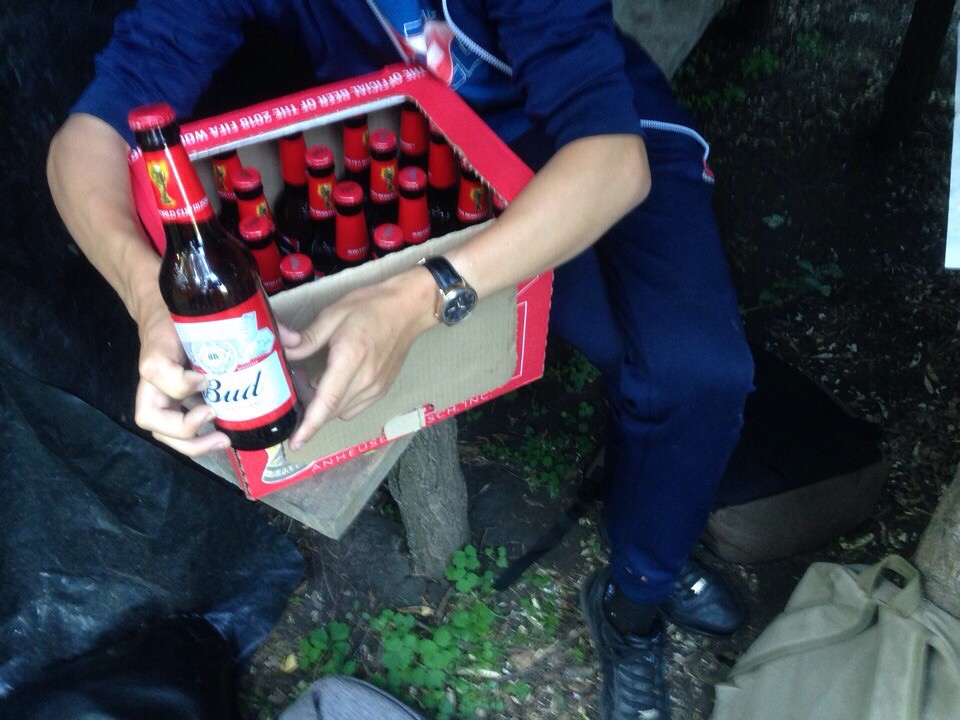In this slightly out-of-focus photograph, a man dressed entirely in navy blue attire - a tracksuit comprising navy blue pants, a sweater, and a t-shirt with an indistinct logo - sits on a rustic park bench characterized by tree bark-like legs and a wooden base. Wearing black trainers, black socks, and a black watch, the man prominently displays a Budweiser beer bottle with a red cap, notable for its brown glass and white label bordered in red that reads "Bud." Next to him, he holds a cardboard box filled with these beer bottles, specifically identified as the official beer of the 2018 FIFA World Cup. At the man's feet are two bags: a grey knapsack and a fallen canvas bag, further hinting at an outdoor setting possibly in a park, evidenced by a nearby trash can.